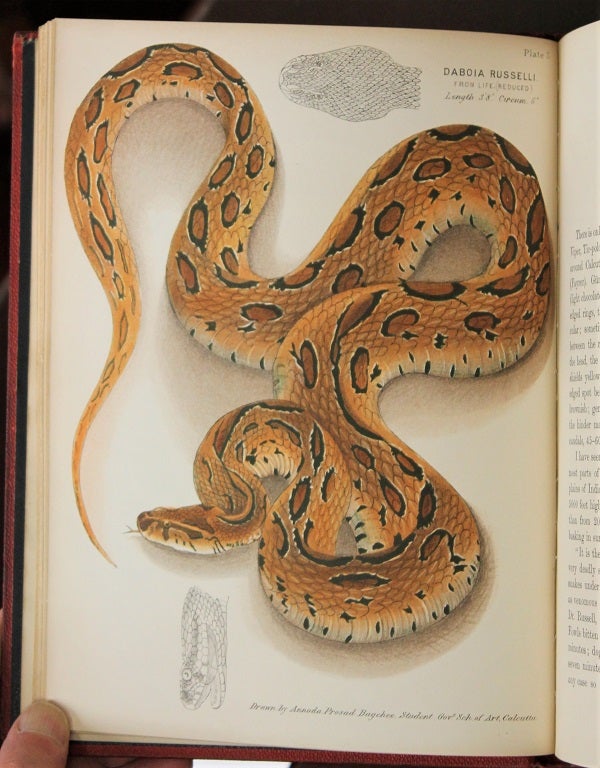The image depicts a detailed, colored drawing of a large snake on a page from a book, held open by a person's thumb visible in the bottom right corner. The snake, labeled "Daboia russelii," showcases an intricate color palette of orange, brown, black, and cream. Its body features deep orange spots with black outlines on the top, and a cream underside dotted with small black marks resembling sesame seeds. The snake is arranged in a zigzag pattern across the page, with its proportionally small head distinguished by a protruding forked tongue and visible nostrils. Additional small sketches, including a top-down depiction of the snake's head, provide further anatomical details. The snake's detailed scales and the S-shaped curls emphasize its length, which would be about three times the page if fully extended.